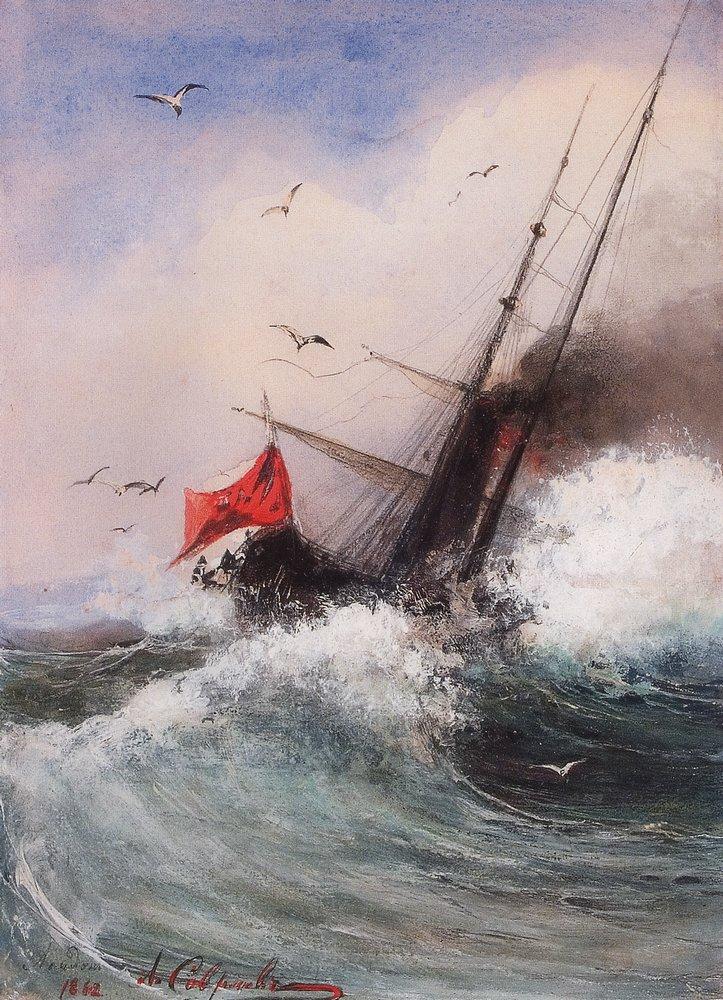This rectangular image, approximately 6 inches tall and 4 inches wide, features a detailed painting of a distressed sailing ship at sea. The bottom half of the ship is black, partially blurred, with its sails lowered, and its mast ablaze, spewing thick black smoke with tinges of red transitioning to gray as it moves to the right side of the image. The ship tilts perilously to the right, as if about to capsize, emphasizing the intense and foreboding atmosphere. A red flag is noticeable on the left side of the vessel's stern. Surrounding the ship, numerous white and black birds, possibly seagulls, are depicted flying above the tumultuous ocean, which is rendered in swirling mixes of blue, green, black, and white. The waves are crashing vigorously against the ship, creating white caps and splashes that add depth and realism to the water. Above, the sky transitions from a soft blue with scattered white clouds to an ominous gray, completing the dramatic and vivid composition. In the lower left-hand corner of the painting, there are indistinct signatures and a date in red, "1882," adding to the historical feel of this powerful and emotive artwork.